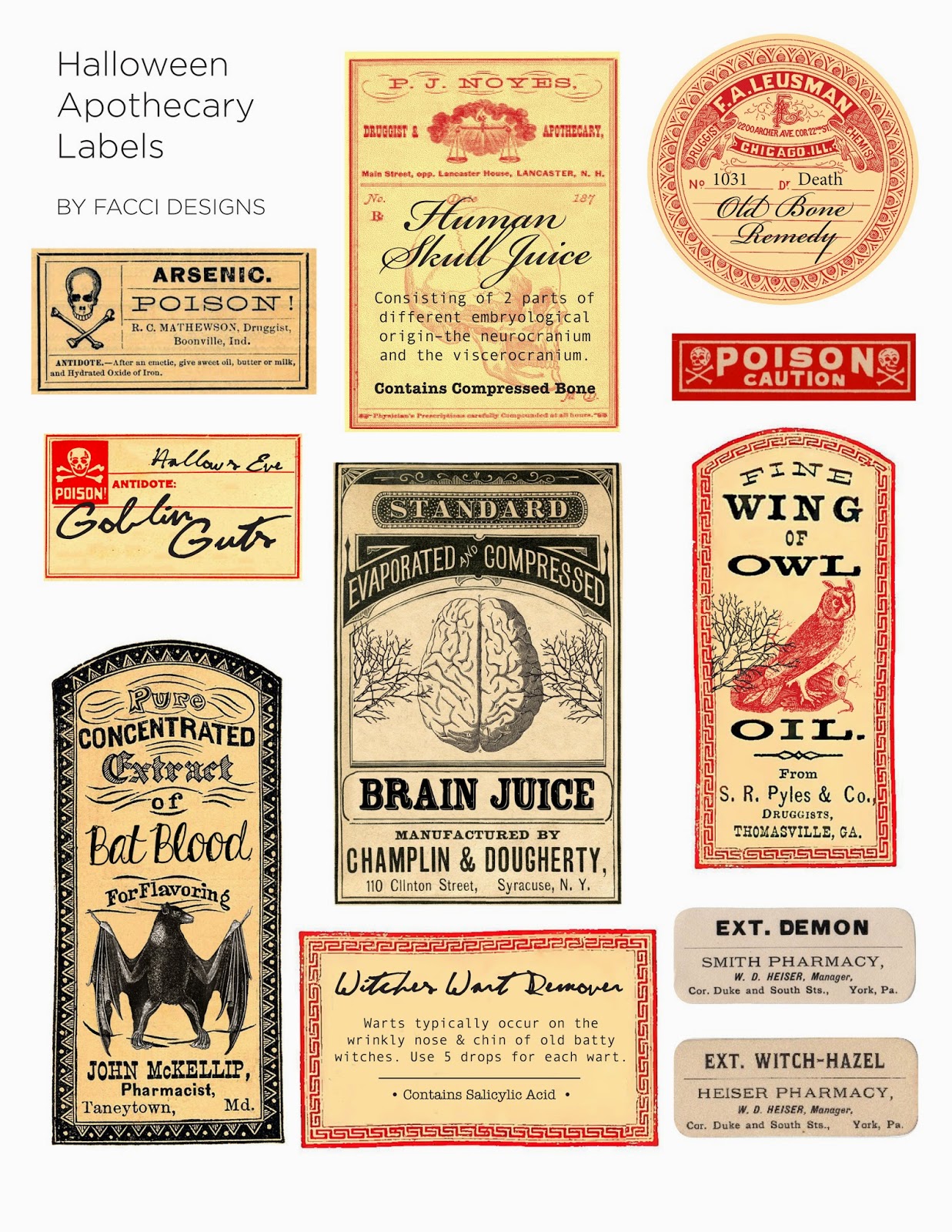The image depicts a collection of Halloween-themed apothecary labels by Facky Designs, shown on an all-white background. At the very top left corner, black text clearly identifies them as "Halloween Apothecary Labels by Facky Designs." These labels are designed to look vintage and weathered, with a spooky aesthetic perfect for Halloween decor or haunted house settings. Each label has an off-white or tan background with black or red text, and some feature drawings of skulls, crossbones, or other eerie imagery.

The top left label is a yellow rectangle with a black skull and crossbones. It reads: "Arsenic Poison. RC Matheson, Druggist, Boonville, Indiana. Antidote: Give sweet oil, butter, or milk and hydrated oxide of iron." Nearby, a label on a red background has a white skull and crossbones and reads "Poison." Another label features the ominous words "Human Skull Juice," detailing that it consists of two different embryological parts: the Neurocranium and the Viscocranium.

Other labels include "Goblin Guts," "Pure Concentrated Extract of Bat Blood for Flavoring," and "Poison Caution." One sinister label reads "Wing of Owl, Oil from C.R. Piles and Co.," decorated with a red owl. Another lists "Evaporated and Compressed Brain Juice," manufactured by "Chaplin and Daughtry, 110 Clinton Street, Siccom, NY."

These intricately designed labels, featuring a mix of white, black, and red colors, are perfect for cutting out and using on bottles or jars to create the ultimate spooky Halloween ambiance.